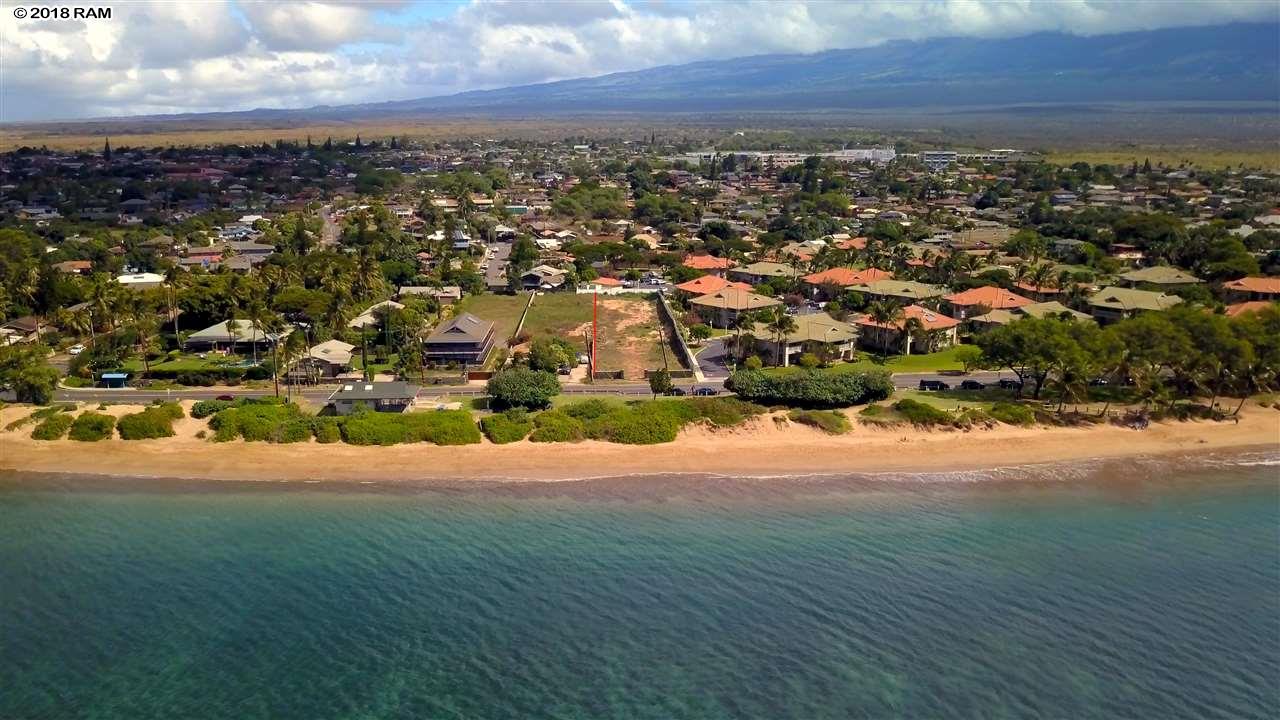This aerial view captures a picturesque beach setting where a long, narrow sandy shore meets the stunning, clear blue waters of the ocean. The beach is bordered by a lush expanse of green vegetation, including bushes and trees, which gradually transition into a multi-lane black asphalt road dotted with moving cars and some parked vehicles. Beyond this road, a quaint town unfolds, with numerous residential buildings sporting orange, green, and grey roofs. The topography rises towards the right side of the image, forming a green-clad mountain. The sky above is a canvas of light blue, interspersed with various white and dark gray clouds, providing a serene backdrop to this vibrant coastal scene. Different shades of vegetation and some open grassy areas, potentially future development sites, further enhance the lively and well-integrated beach town ambience.